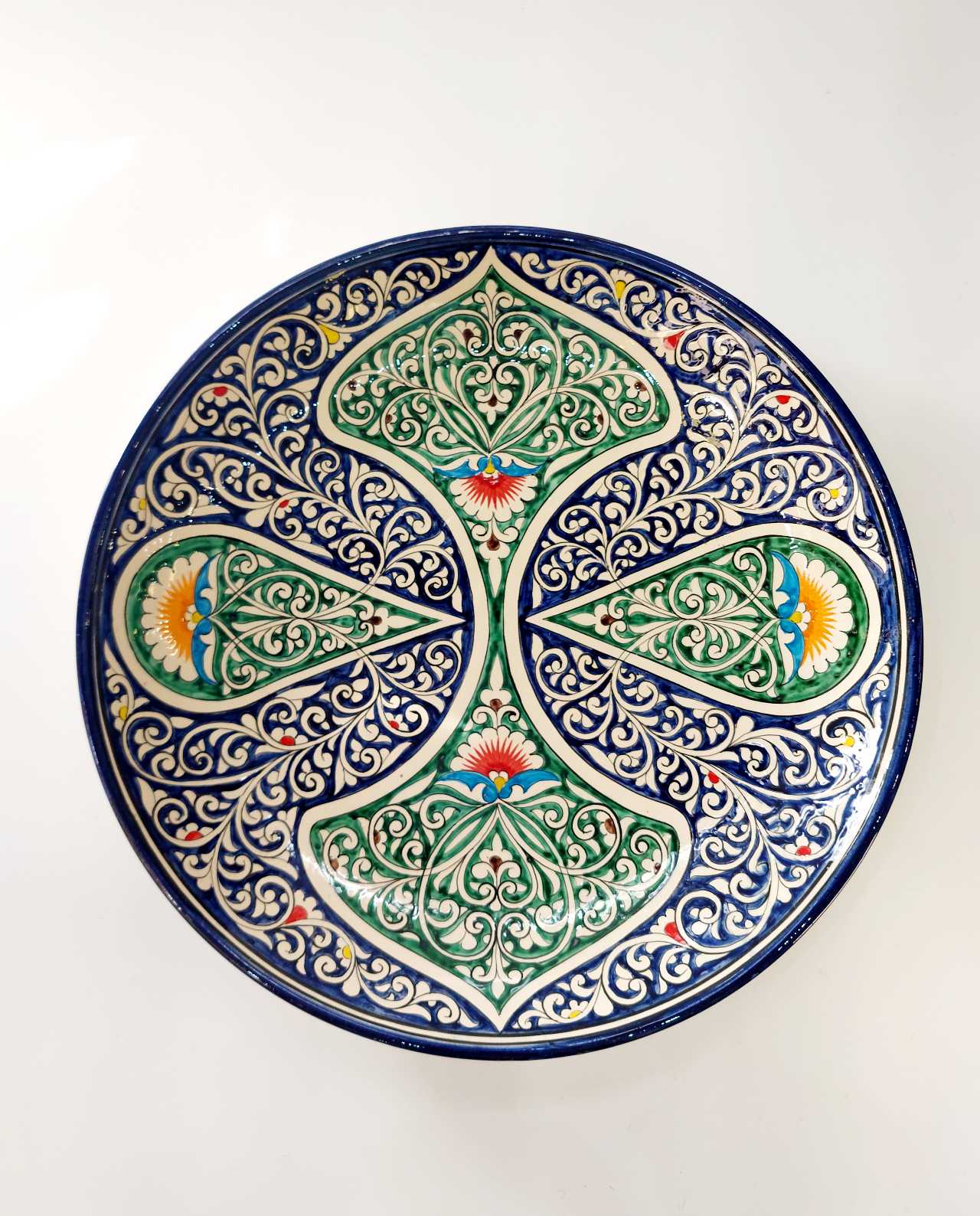The image showcases an intricately decorated, shallow porcelain plate photographed from above, featuring a design reminiscent of Central American or Mexican motifs. The plate's background is a dark navy blue, with ornate white scroll work overlaying it. Central to the design are symmetrically positioned spade-like and teardrop shapes, edged with green and adorned with detailed red and yellow flowers. These shapes are connected in the middle, forming a harmonious pattern. The plate, which appears thick and robust, rests on a tan surface streaked with white, highlighting the vibrant and artistic hand-painted details.